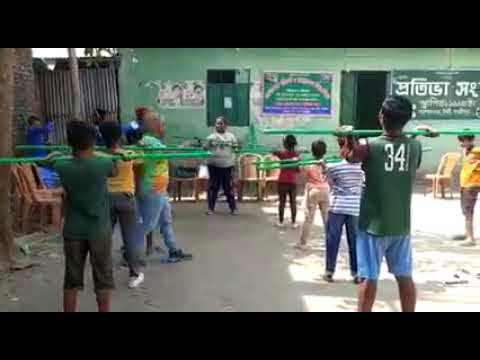In this image, we see a group of children standing outdoors in a courtyard, organized into rows while holding long green rods at shoulder level with both hands. There are about eight children present, arranged in two or three rows, with boys and girls participating. They appear to be involved in an activity similar to a weightlifting class, with one child in the middle demonstrating the action, possibly under the supervision of a couple of adults. The background includes a green building adorned with signs in an unreadable script, which suggests the setting might be in a region like the Middle East. The area features a mixture of brick walls and what looks like corrugated steel paneling, with chairs lining the walls. The ground is sandy, and there is also a tree visible on the left side of the image.